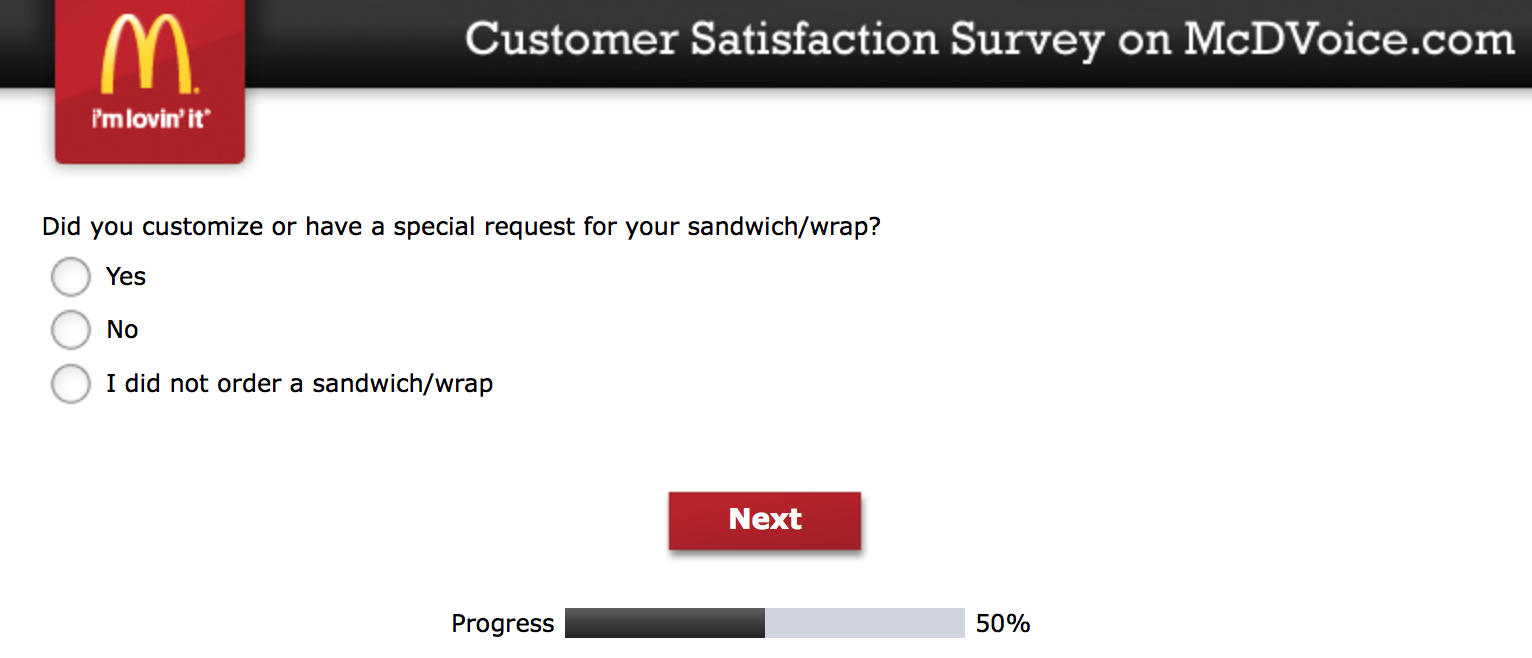This image, sourced from the McDonald's website, features the iconic McDonald's logo positioned on the upper left-hand side. The logo, a bold yellow "M" set against a red background, also includes the tagline "I'm loving it" in white text beneath it. This logo slightly overhangs from a black bar that stretches horizontally across the image.

In the black bar, large white font reads, "Customer Satisfaction Survey on mcdvoice.com." Beneath this bar, the background transitions to white, where a survey question is prominently displayed in black font: "Did you customize or have a special request for your sandwich/wrap?" Three response options are available: "Yes," "No," and "I did not order a sandwich/wrap." Toward the bottom of the image, a "Next" button is visible above a progress bar indicating that the survey completion is at 50%.